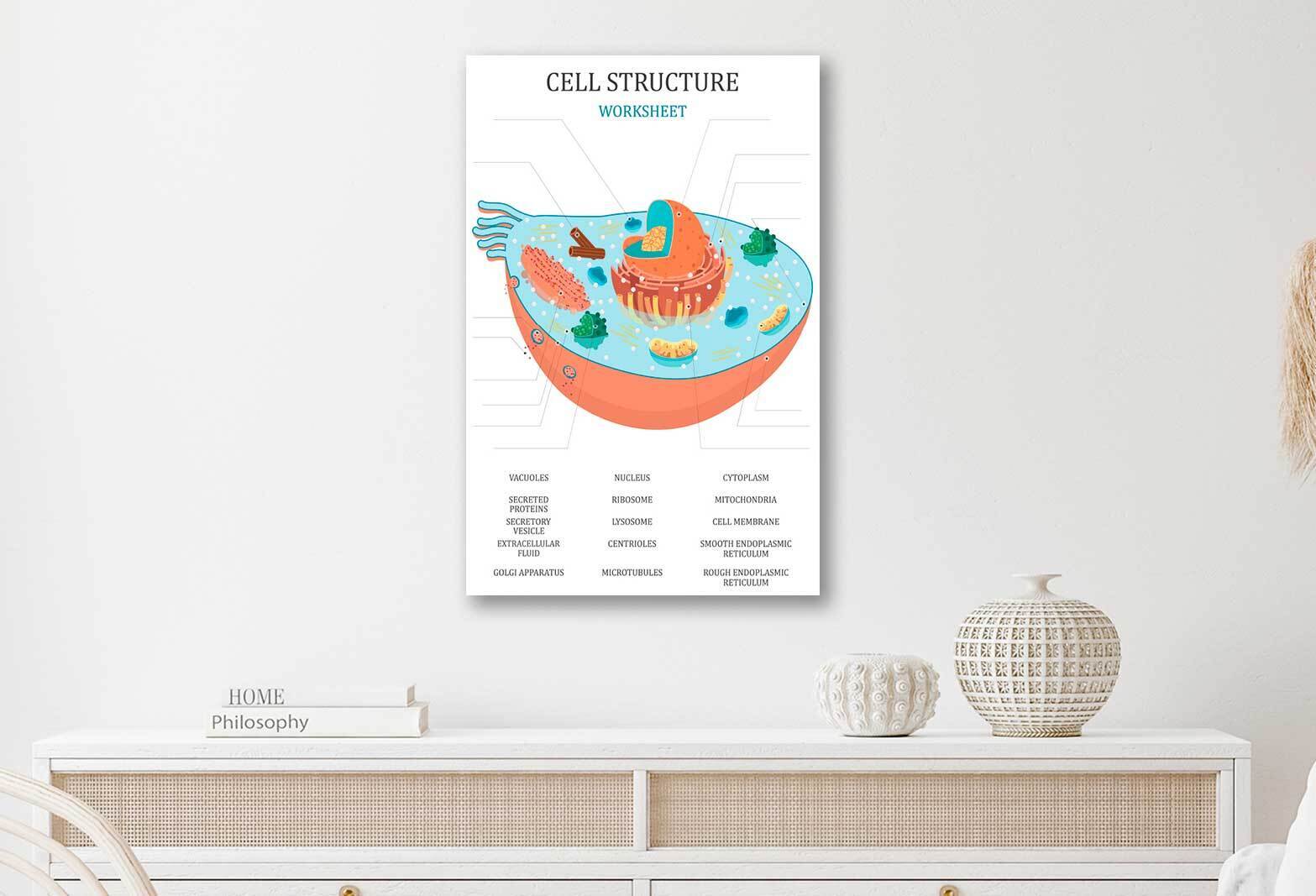This interior photograph captures a minimalist, predominantly white room. The focus is on a wide, white dresser occupying the bottom of the image. The dresser features two visible drawers with golden handles and a detailed finish above them, as well as a subtle brown mesh pattern on top. Adorning the top of the dresser are two white sculptures—a small cactus and a plump vase—alongside two horizontally placed books titled "Home" and "Philosophy".

Off to the side, the top of a white chair is faintly visible. The background showcases a stark white wall adorned with a vertical poster titled "Cell Structure Worksheet" at its center. The poster details a 3D illustration of a cell, complete with an array of arrows and labels pointing to various components of the cell. Though some text is too small to read, it appears to serve as an educational tool for identifying parts of the cell, with sections color-coded in shades of blue, green, teal, and orange. Overall, the scene exudes a clean, scholarly ambiance through its cohesive white theme and subtle educational elements.